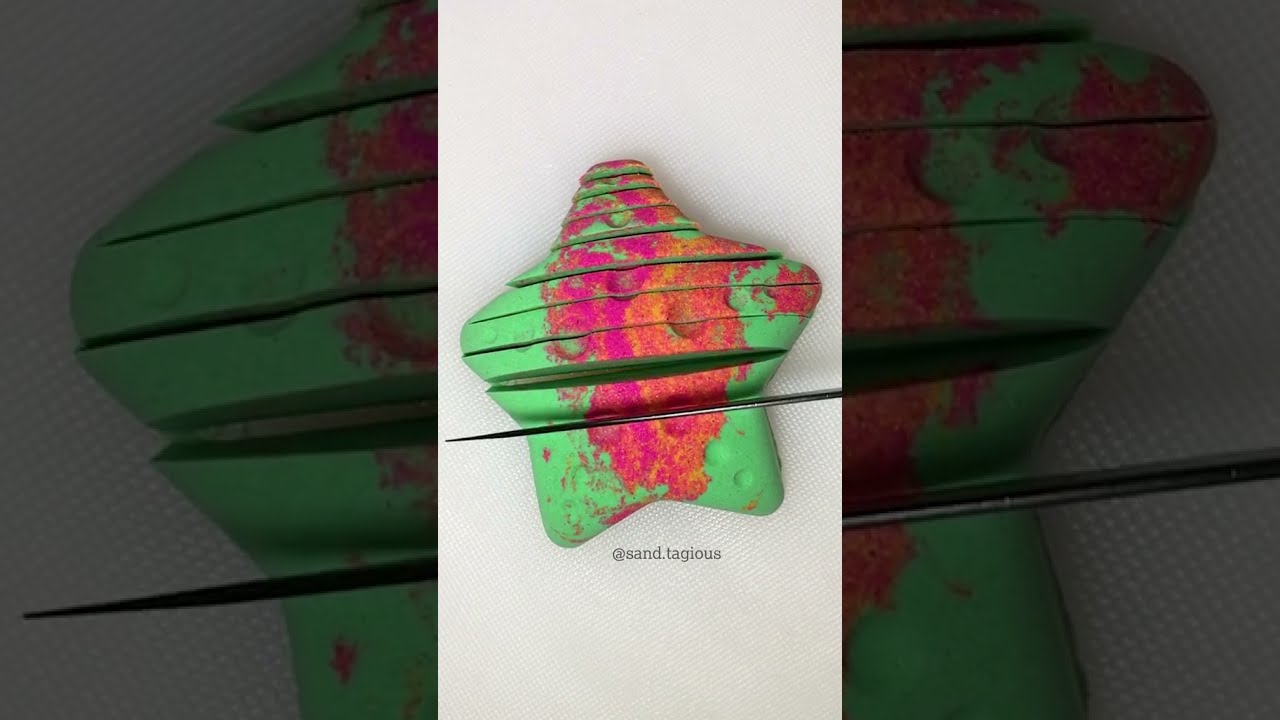The image is a horizontally rectangular, three-panel photograph featuring a star-shaped object, primarily green with craters and accents of pink, orange, purple, and yellow. The central panel, which is much brighter than the darker left and right panels, shows the star being horizontally sliced by a knife or blade, leaving thin slices from top to nearly two-thirds down the star. This star-shaped item, possibly made from play-doh, clay, or even cookie or cake dough, is set on a white surface resembling a plastic cutting board. The left and right panels provide close-ups of the star from different angles but are significantly darker. The image caption at the bottom reads "at sand Tejas."